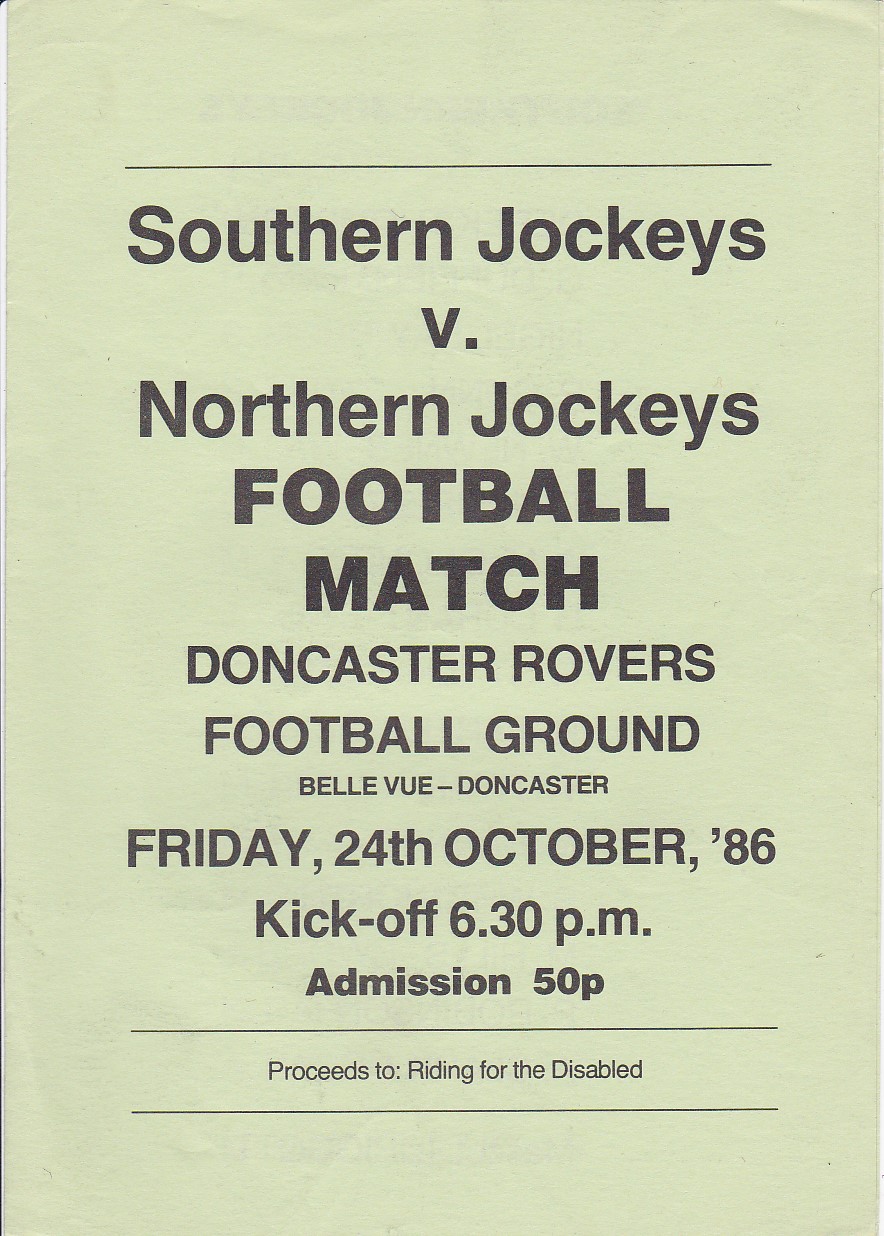This image features a simple, yet eye-catching informational flyer for a football match. Printed on light, pale green paper, the flyer announces a game between the Southern Jockeys and the Northern Jockeys in bold, capitalized black font. Below this, it specifies that the match will take place at the Doncaster Rovers Football Ground, located at Bellevue, Doncaster. The details continue with the date and time of the match: Friday, 24th October, 1986, with kickoff at 6:30 PM. Admission is listed as 50p. The flyer also includes two thin horizontal lines, between which it states that proceeds from the event will benefit "Writing for the Disabled." The clean, straightforward design of the flyer suggests it is intended for quick public dissemination, such as posting on walls or utility poles to attract attendance and support for the cause.